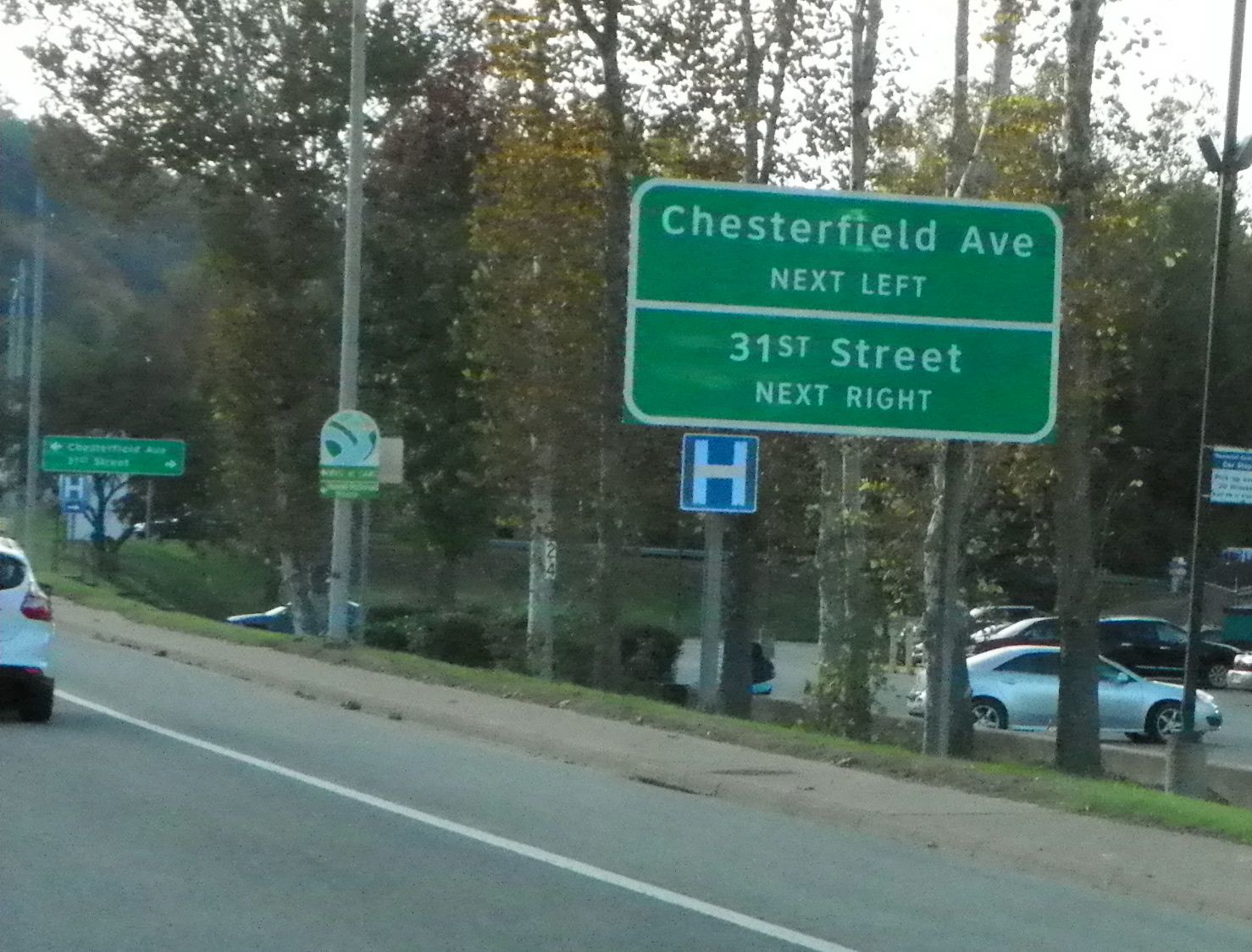A busy roadway likely designated as a route, not a freeway, stretches across the image, bordered by a sloping hill on one side. Nestled at the base of this hill is a parking lot featuring a red and a silver car. A sidewalk runs along the side of the road. Prominently positioned in front of a dense cluster of trees descending the hill, a green sign with white lettering reads "Chesterfield Avenue, next left" and "31st Street, next right." Below this sign, a blue "H" symbol indicates a nearby hospital. The sign repeats further down, detailing the upcoming splits. In the bottom left corner of the image, a white car, positioned just north of a white Kia, is visible near the breakdown lane and adjacent sidewalk.